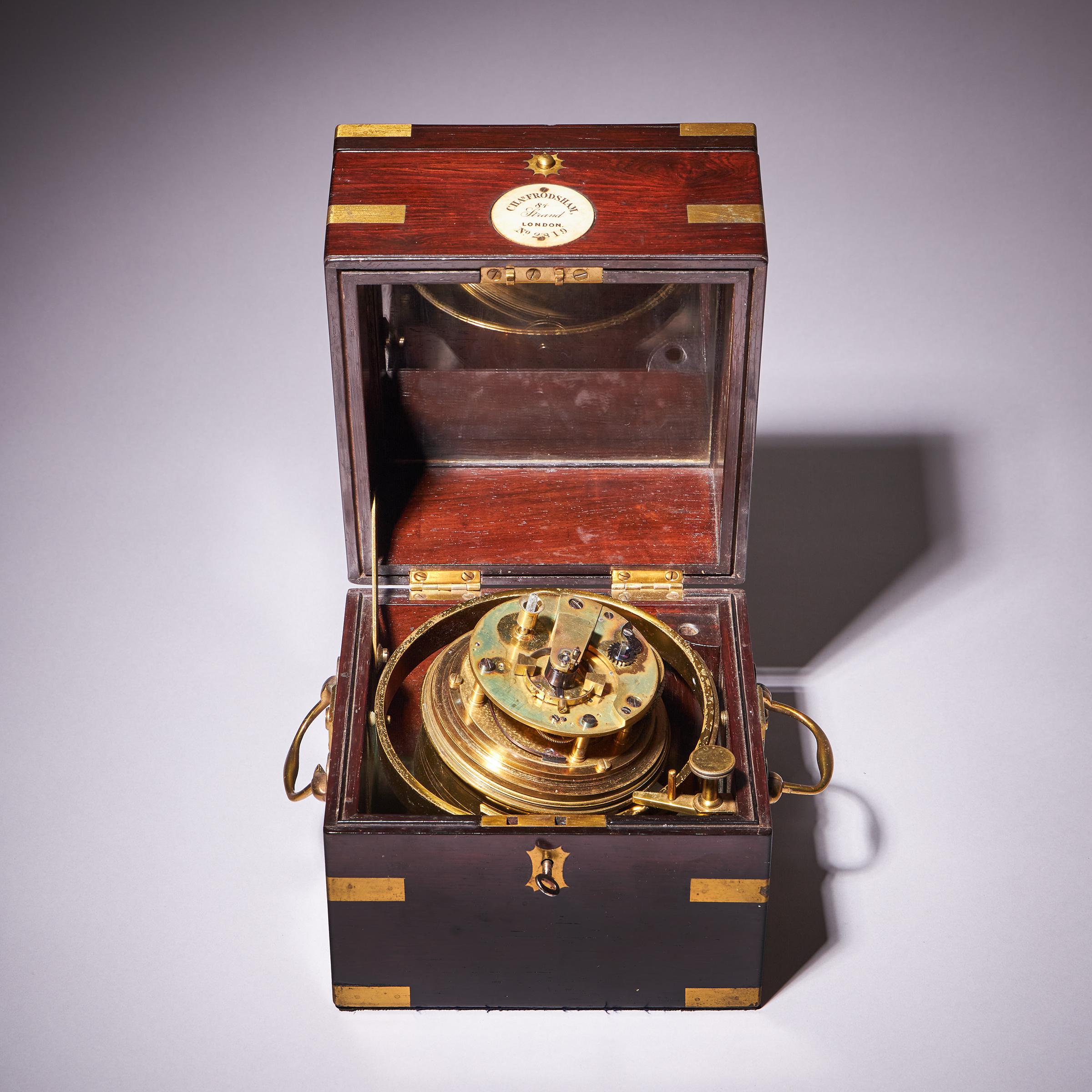The image depicts an antique wooden box with ornate brass and gold-colored fittings, suggesting a vintage electronic or mechanical device. The box, constructed from a reddish-hued wood, opens upwards to reveal its intricate contents. Inside the lid, there is a mirror that reflects a central mechanism composed of concentric golden circles, resembling the components of a telescope or possibly a musical apparatus. This central mechanism includes a brass handle on either side and a cylindrical key situated at the front. The box also features two golden side handles, indicating it is portable. An inscription on the top, possibly reading "Crendleshaw," hints at its origin or manufacturer, and it is noted to be made in London with a model number that appears to be 16 or 19. The piece is both functional and decorative, set against a stark white background that emphasizes its vintage craftsmanship and aesthetic detail.